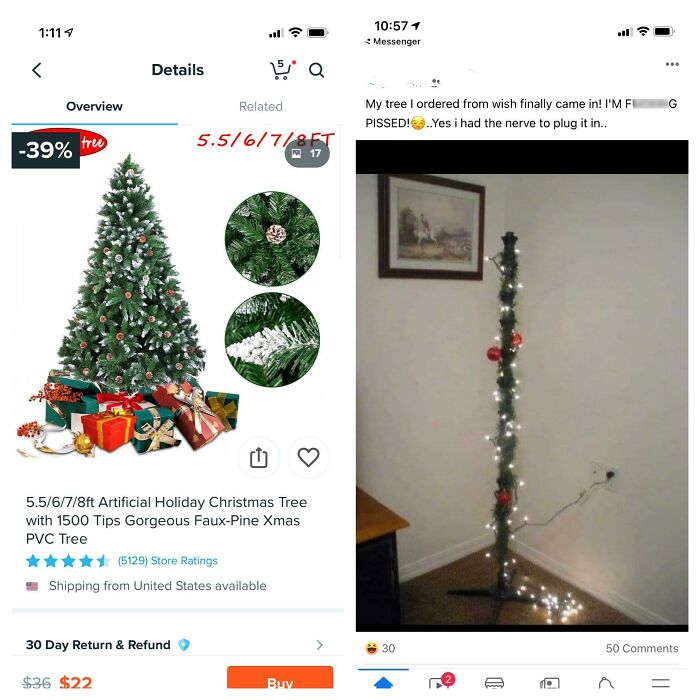Certainly, here's a refined and detailed caption for the described image:

---

**Side-by-Side Image Description:**

*Left Image:*

- **Background**: White
- **Device Display**:
  - **Time**: 1:11, displayed in the top center
  - **Wi-Fi Indicator**: Three out of four bars filled, indicating good Wi-Fi reception
  - **Battery Icon**: Appears fully charged
  - **Arrow Icon**: Black, pointing towards the right
  - **Details Section**: Includes a black magnifying glass icon next to the word "Details"
  - **Notification Badge**: Red circle with the number '5'
  - **Tabs**: Two tabs labeled "Overview" (highlighted and underlined) and "Related"
  - **Product Details**: 
    - **Description**: "Artificial Holiday Christmas Tree with 1,500 tips"
    - **Sizes**: 5.5/6/7/8 feet
    - **Design**: "Gorgeous for old pine Xmas PVC"
    - **Rating**: Almost 4.5 stars, in blue text
    - **Reviews**: 5129 reviews, store ratings indicated in blue
    - **Shipping**: From the United States
    - **Price**: $22, indicated in orange

*Right Image:*

- **Description**: A personal post or message
  - **Message Content**:
    - Opening line: "My tree out, what if a wish finally came in?"
    - Expresses frustration using blurred out expletive: "I'm F-ing pissed"
    - Describes personal experience: "Yes, I had the nerve to plug it in, and it looks like a stick. It's not even a tree, just a stick with lights."

---

This caption provides a comprehensive and detailed description of each image, making it clear what each element in the images represents.